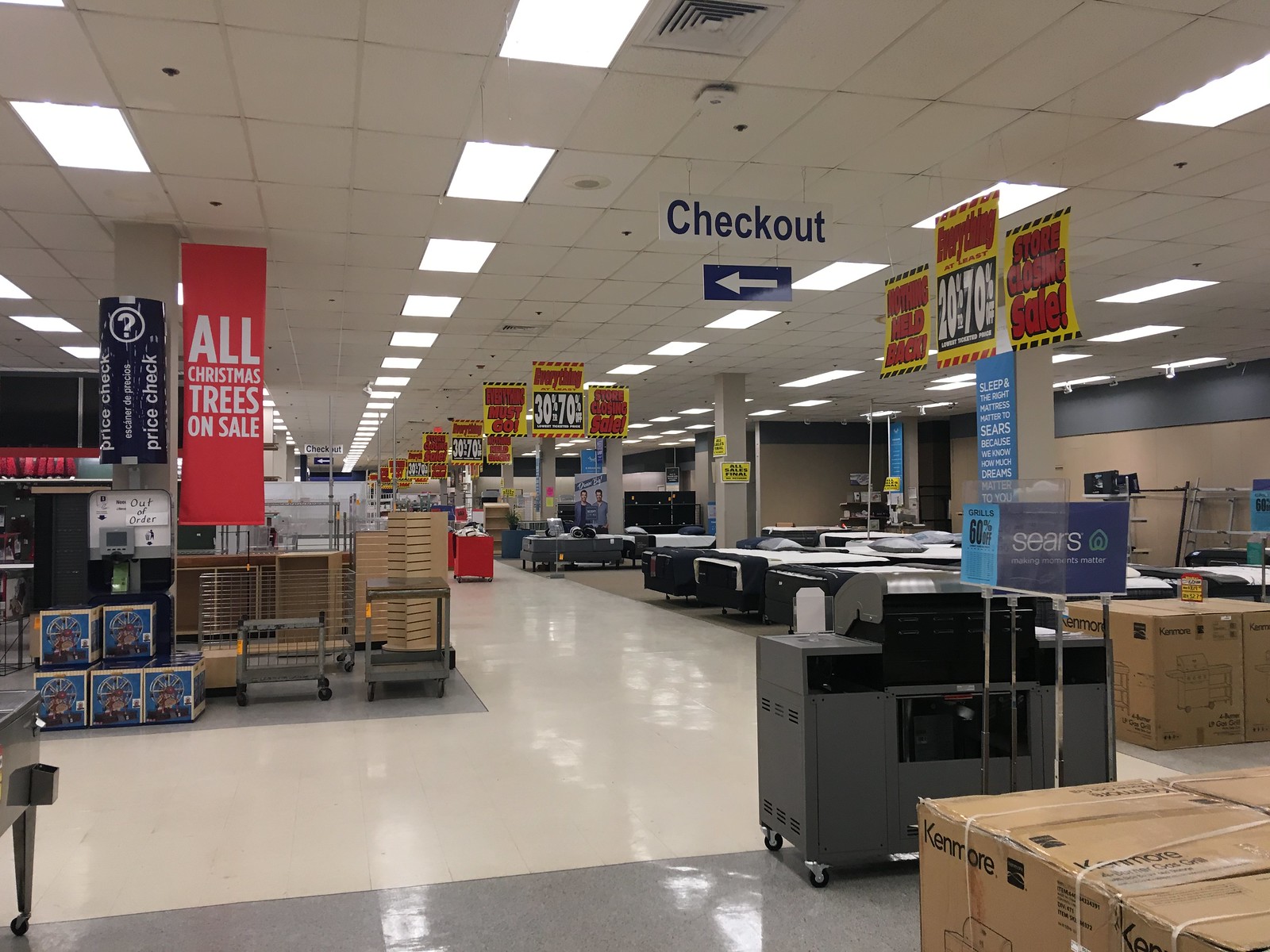The photograph captures the interior of a retail store, focusing down an aisle. The floor features a polished white tile with a gray border, reflecting the store's well-maintained appearance. The ceiling is a white drop style, interspersed with illuminated squares. Centrally placed within the frame is a clear sign with the words "Check Out" in blue letters, accompanied by a solid white arrow pointing to the left; the arrow is thick and enclosed in a rounded rectangular shape. 

In the bottom right corner of the image, the tops of several boxes are visible, alongside what appears to be the back of a small grill, which is gray with a black top. The top of the grill is just visible peeking over the edge of the shelf.

On the left side of the aisle, a large rectangular sign hanging from the ceiling announces a sale: "All Christmas Trees On Sale" in prominent white text against a red background. Additional red signs with white writing can also be seen hanging from the ceiling, reinforcing the festive promotional display.